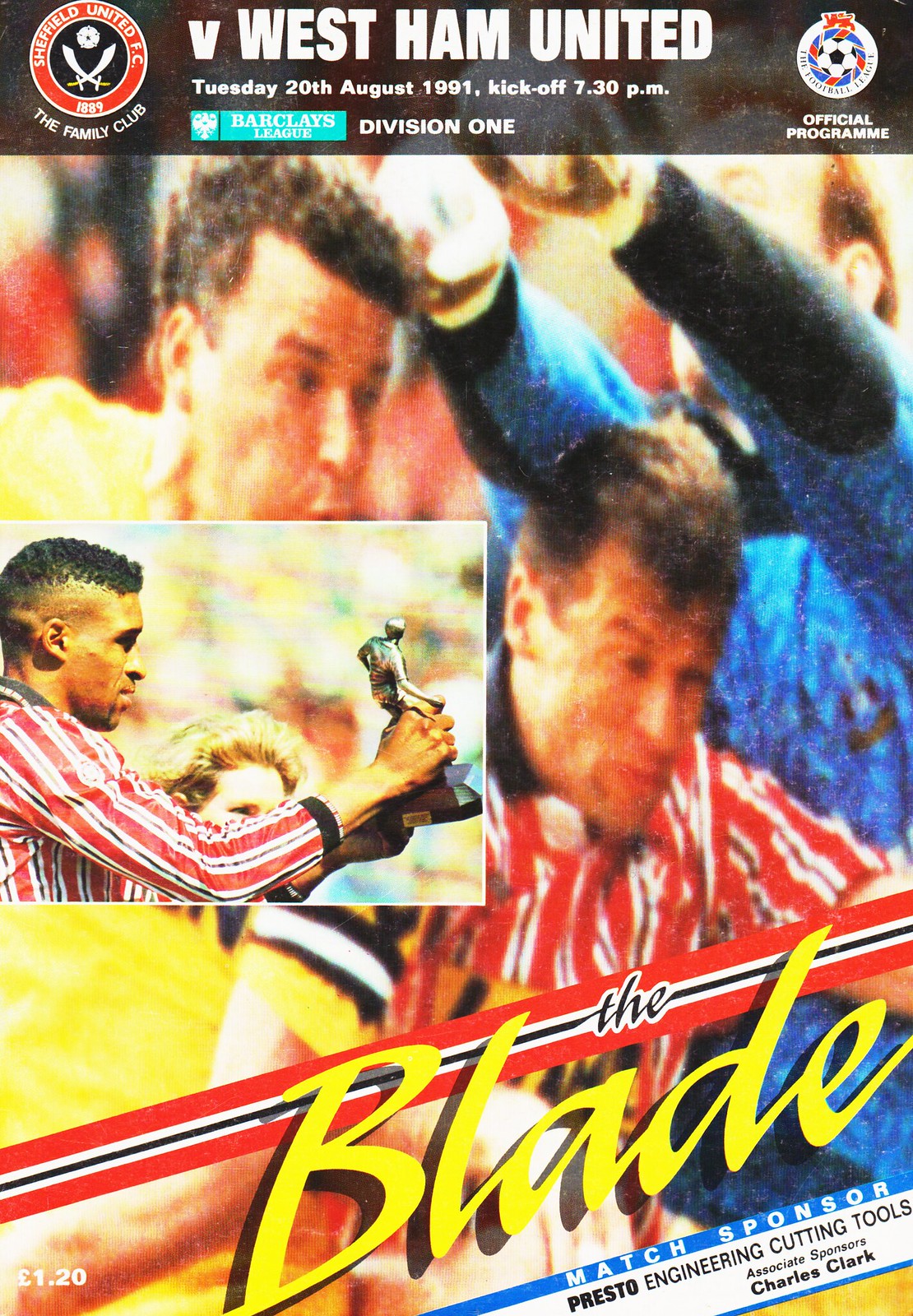This image is a vintage cover of an official soccer program from a match between Sheffield United FC and West Ham United, held on Tuesday, 20th August 1991, with a kickoff at 7:30 p.m. The program prominently features several elements: 

At the top, a black bar with white letters reads "Sheffield United FC - The Family Club." Directly underneath, it states "West Ham United" and "Barclays League Division 1." 

The main background is a faded, somewhat blurry collage of soccer action, showing three players, two of whom are in distress, with short hair and wearing yellow and red jerseys, against a backdrop that suggests a crowded stadium.

Superimposed on the left-center of this backdrop is a clear, squared section featuring a young African-American man wearing a red and white striped long sleeve jersey. He holds a trophy aloft in his right hand, exuding a sense of triumph.

On the right side of the cover, there are logos, including one of a soccer ball and seal, with the text "Official Program." At the bottom in large, diagonal yellow letters, it says "The Blade," followed by details on the match sponsor "Presto Engineering Cutting Tools" and associate sponsor "Charles Clark." The bottom left corner mentions the price of £1.20.